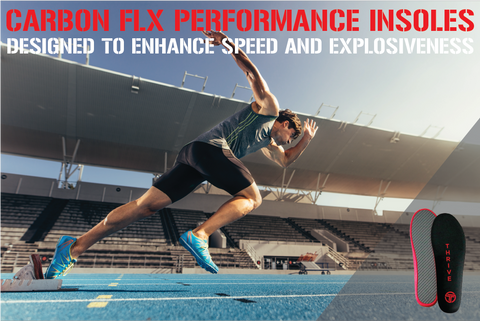This detailed photograph captures a professional male runner at the starting blocks on a blue track under a clear daytime sky in an empty stadium. The athlete, who appears Caucasian with brown hair and clad in a gray tank top, tight black shorts, and blue sneakers accented with yellow threading, is seen in mid-action. His left foot is pressed against a metal foot pad to aid in his explosive start, while his right knee is bent and his right foot is lifted, emphasizing his readiness to sprint. The track, with its white lines and coarse texture, extends across the bottom of the rectangular image. Red text at the top reads "Carbon FLX Performance Insoles," followed by a white subheader, "Designed to Enhance Speed and Explosiveness." In the lower right corner of the photograph, two products are superimposed: a black insole bearing the word "Thrive" in red print and a gray insole outlined in red. The stadium seats remain vacant, and the overall composition, including the professional setting and product placement, suggests this image is part of an advertisement promoting these performance insoles.